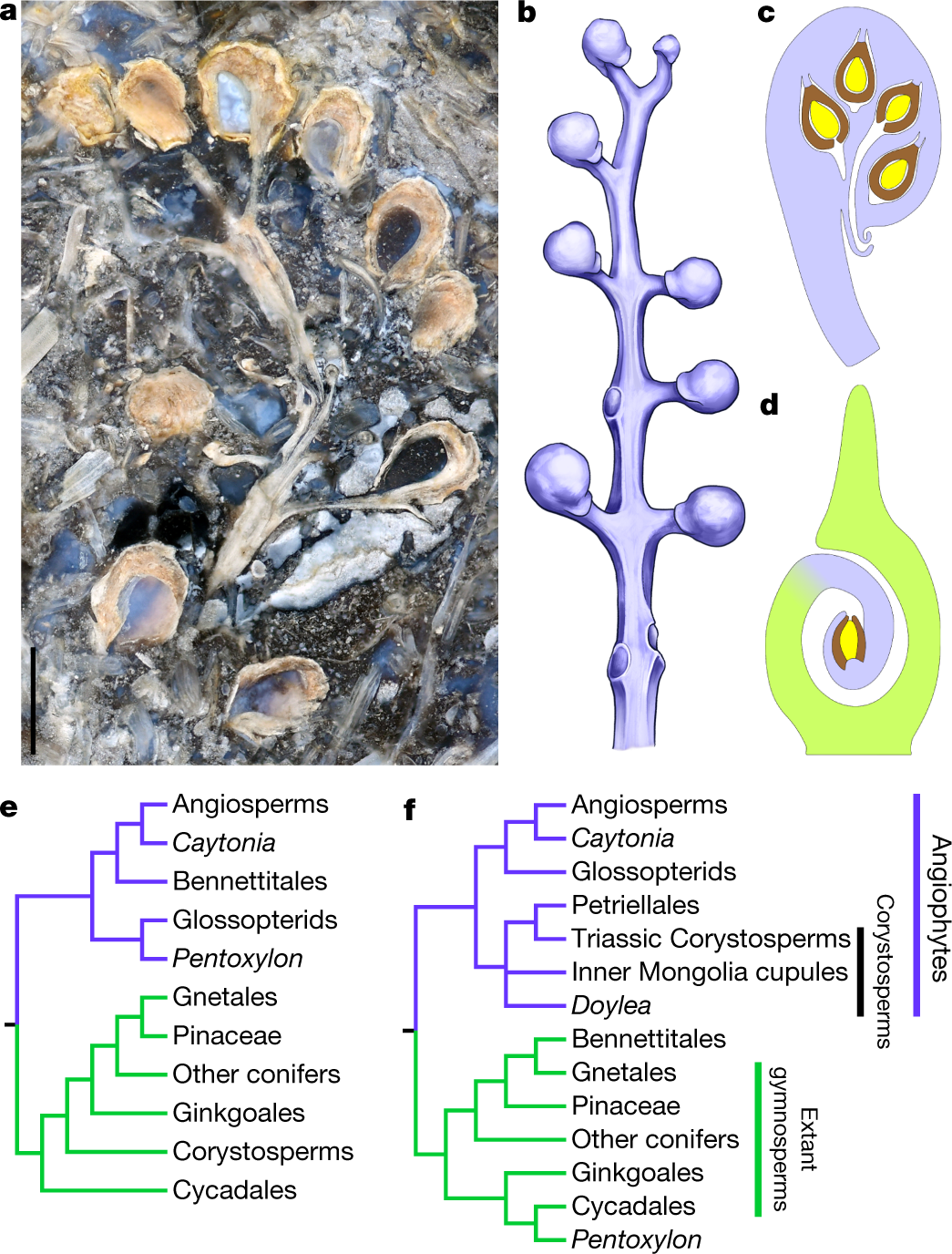The image is a detailed scientific infograph categorizing various images labeled A through F. It begins with section A, which features a real-life, outdoor photograph of a biological specimen, possibly a plant, preserved in nature. This specimen is connected to water and appears complex with multiple elements attached to it. Sections B, C, and D are fully illustrated and resemble textbook diagrams, providing detailed views of the same plant structure depicted in A. These illustrations use colors such as lavender for the plant's stalk and nodules. 

Sections E and F introduce the categories "Angiophytes," "Choriosterberms," and "Extant Gymnosperms," organizing them in a taxonomy format with lines converging to connect related items. The images include a part that displays a purple stem with circular structures and a side view with yellow and orange circular nodules, along with a front view in light green that forms a swirl pattern. Text annotations and bracket formats elucidate the connections between these various parts and categories, highlighting the intricate taxonomy and relationships within this plant family. Overall, the infograph merges actual biological specimens with detailed illustrations and scientific classifications, underscoring its educational purpose related to biological and botanical studies.